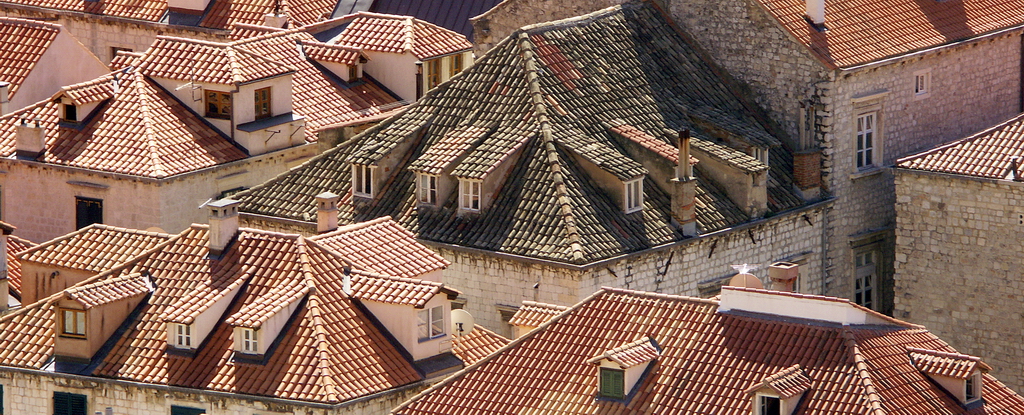The image captures a dense cluster of rooftops in what appears to be a European village, viewed from a high vantage point. The scene is dominated by rows of closely packed buildings, all featuring uniformly tan-brown, small square tiles arranged in horizontal rows. Many of these rooftops have small windows jutting out, also covered in the same tiles and adorned with a mix of shutters and various window styles, some crosshatched and some with two panes.

In stark contrast, the central building features a weathered, larger roof made of similarly styled tiles that are mainly greenish-black with patches of red, lending it an aged and different appearance compared to the surrounding rooftops. This central roof, like the others, comes to a long point down its center. Additionally, on the right-hand side of this central building, there is a structure with a flat roof that stands out amidst the otherwise uniformly pitched roofs. The buildings below the roofs exhibit a variety of architectural touches, including white, gray bricks, and even cobblestone facades, evoking a sense of historical charm and antiquity. Overall, the captivating detail and varied textures convey a rich impression of an old European village scene.